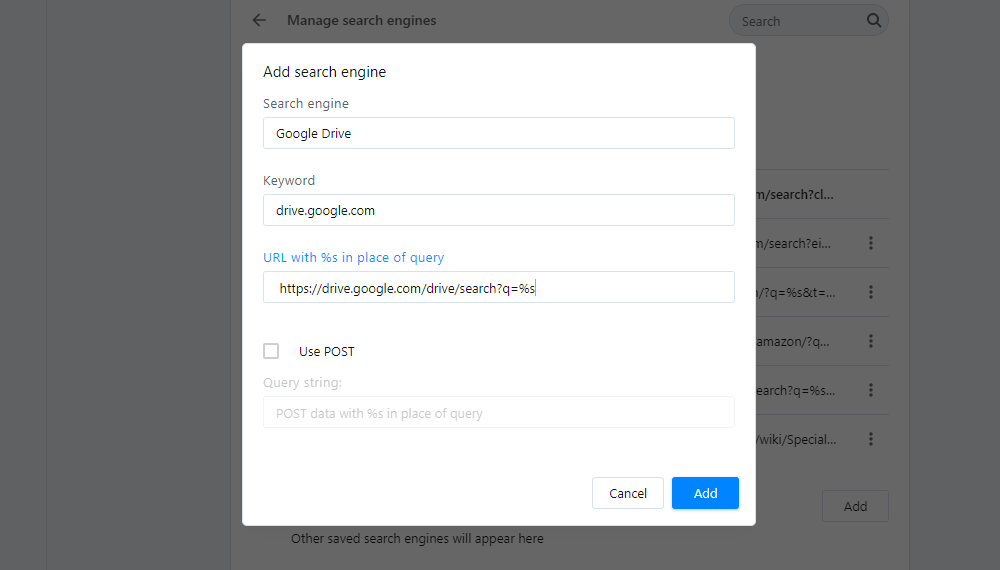Detailed Image Caption:

The image displays a web page overlaid with a semi-transparent gray shade, indicating an active pop-up window. The main page in the background features a navigation header. On the left, a left-facing arrow labeled "Manage search engines" is visible. Toward the right end of the header, there's a search box with a magnifying glass icon. Below the header is a list consisting of six lines, each ending with a horizontal three-dot menu. At the bottom of this section, an "Add" button is present. In the bottom left corner, text states that "Other saved search engines will appear here."

In the foreground, the pop-up window titled "Add Search Engine" is prominent. It contains multiple input fields and instructions. The first input field is labeled "Search Engine," with the value "Google Drive" inside. Directly below this is another label, "Keyword," accompanied by an input box containing "drive.google.com." Underneath, in sky-blue text, it reads "URL with %s in place of query," followed by an input field containing the URL: "https://drive.google.com/drive/search?q=%s," and the cursor is blinking at the end of this URL, also in sky blue.

To the right of this URL input field is a checkbox labeled "Use POST." Below this section, further instructions state "Query string," with another input box containing the text "post_data=%s."

At the bottom of the pop-up, there are two actionable buttons: "Cancel" and "Add."